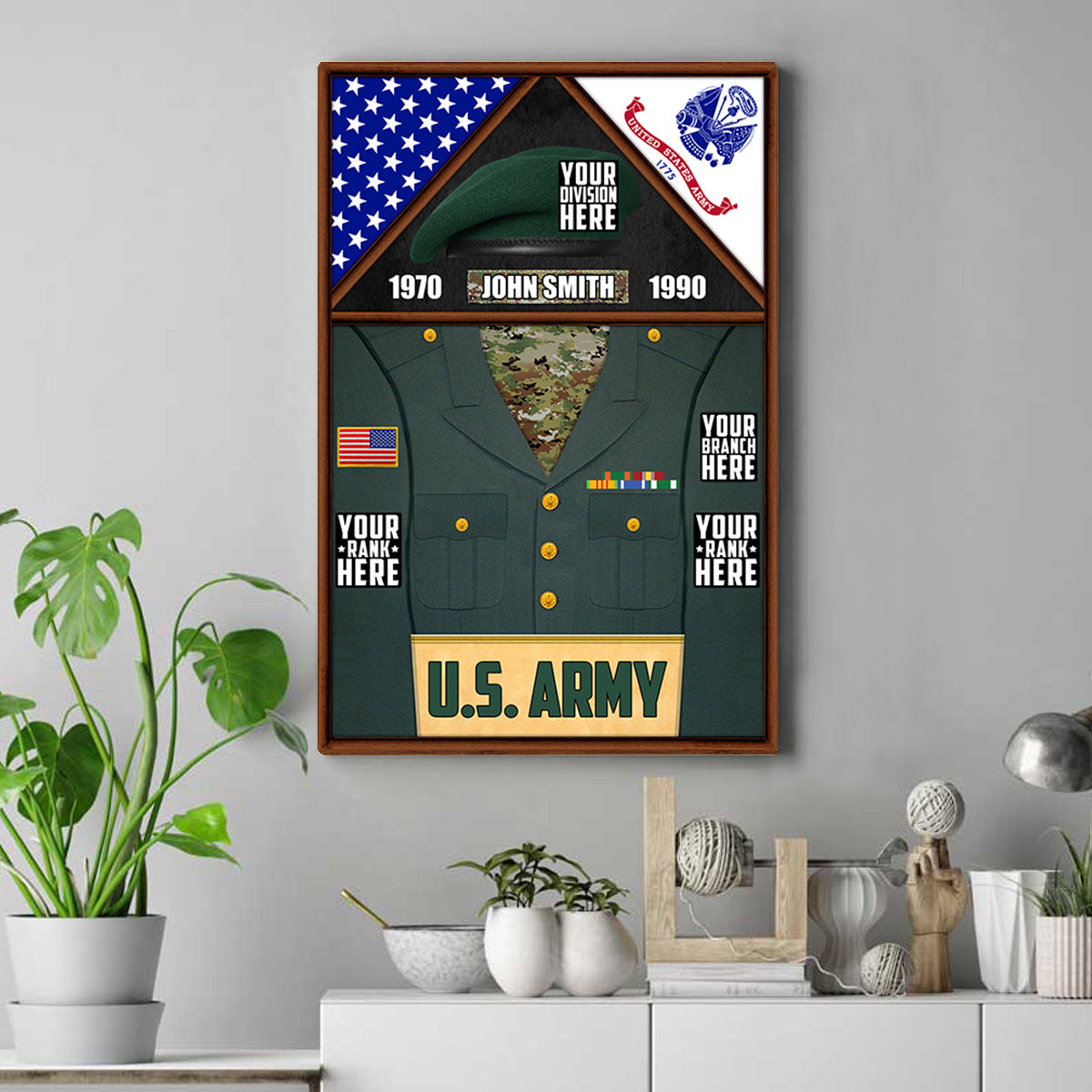This is a color photograph capturing the interior of a cabin, showcasing a framed poster on a light gray wall. The poster, positioned centrally, displays a U.S. Army dress uniform, complete with medals over one pocket, and an American flag patch on one shoulder. It features placeholder text on the arms for "your rank here" and "your branch here," with a military cap and the name "John Smith." The years "1970" and "1990" flank the image, signifying the period of service. At the top, three triangles, representing folded American flags, are to the left, while the U.S. Army insignia is to the right.

Beneath the framed poster, the cabin wall has white shelves adorned with various decorative items, including bowls of yarn, twine, and white sculptures. A Monstera plant in a white pot is positioned to the left of the shelves. The background wall is light gray, enhancing the contrast and highlighting the framed military memorabilia at the center.